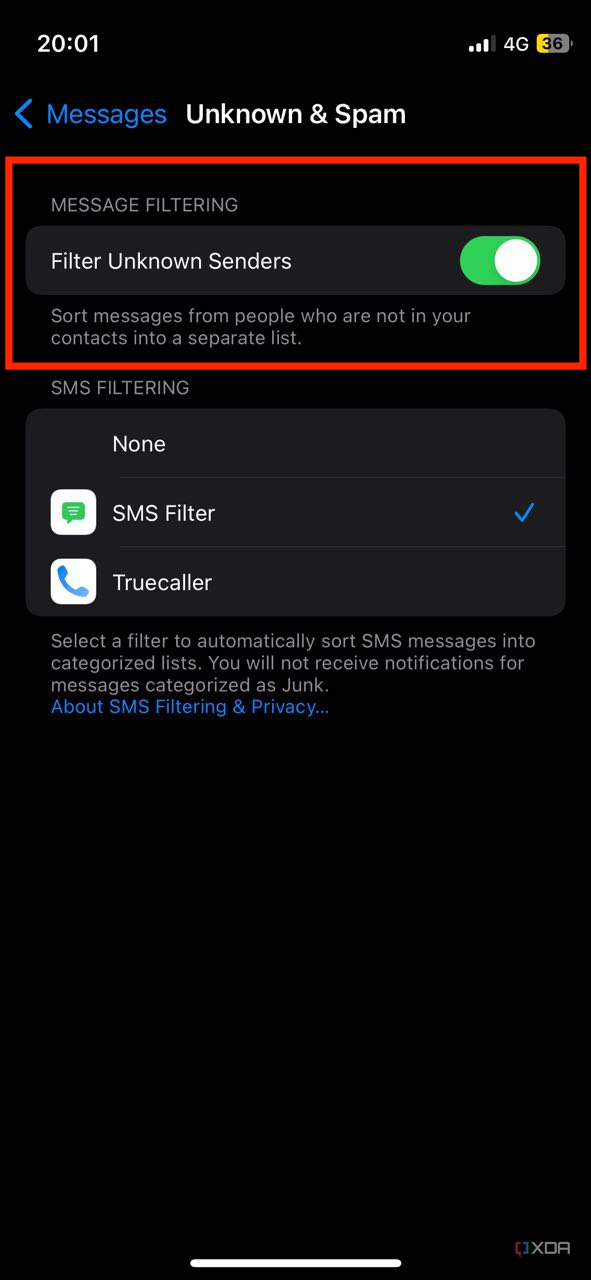The image showcases the screen of a mobile phone. On the top-left corner, the year "2001" is displayed, accompanied by signal bars, a "4G" symbol, and a battery icon indicating 30% power, shown in yellow. Below this status bar, there is a blue header labeled "Messages" with a left-facing arrow, also in blue. Underneath, the screen reads "Unknown" and "Spam" with the text "Message filtering" beneath them. 

A toggle for "Filter Unknown Senders" is turned on, indicating that messages from contacts not saved in the phone's address book will be sorted into a separate list. This entire section is outlined by a red rectangle.

Further down the screen, there's an option for "SIMs Filtering," which is apparently set to "None." However, another checkbox is labeled "SIMs Filter" and is marked as "Checked" with the status "Yes." Next, a "True Call Caller" option is visible.

The instructions below provide information on selecting a filter to sort SMS messages into categorized lists, noting that notifications for messages identified as junk will not be received. There is a blue link labeled "About SMS filtering and privacy."

The background of the phone's screen is predominantly black, with a slate gray section. The bottom-right corner of the screen has the text "Q XDR," and the middle-bottom section shows a white line. The primary colors used throughout the screen are yellow, white, blue, red, and green.